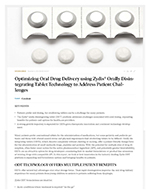This image features a pharmaceutical advertisement emphasizing the benefits of a specific drug, presumably named Xylee Oralee. Central to the visual is a prominently focused blister pack, crafted from a sleek silver material, containing four round, white tablets. These tablets are meticulously placed directly in front of their respective slots in the blister pack, drawing immediate attention to their form and consistency.

Above the blister pack, in bold black lettering, the headline reads, "Optimizing Oral Drug Delivery Using Xylee Oralee." This headline sets the theme for the advertisement, although the finer details of the accompanying article remain out of focus and unreadable, likely due to the minimization of the text in the image.

Beneath the headline, the structure of the article is suggested by additional bolded black text delineating key points. There is a clear outline indicated by four bullet points under the headline, which likely summarize the crucial aspects of the drug's benefits or usage instructions. Following these bullet points, there are paragraphs of text that provide further elaboration, although their exact content is not discernible from the image.

The overall composition of the advertisement ensures the blister pack and the tablets are the primary focus, highlighting the tangible product while alluding to the detailed, though de-emphasized, informational content provided in the textual sections.